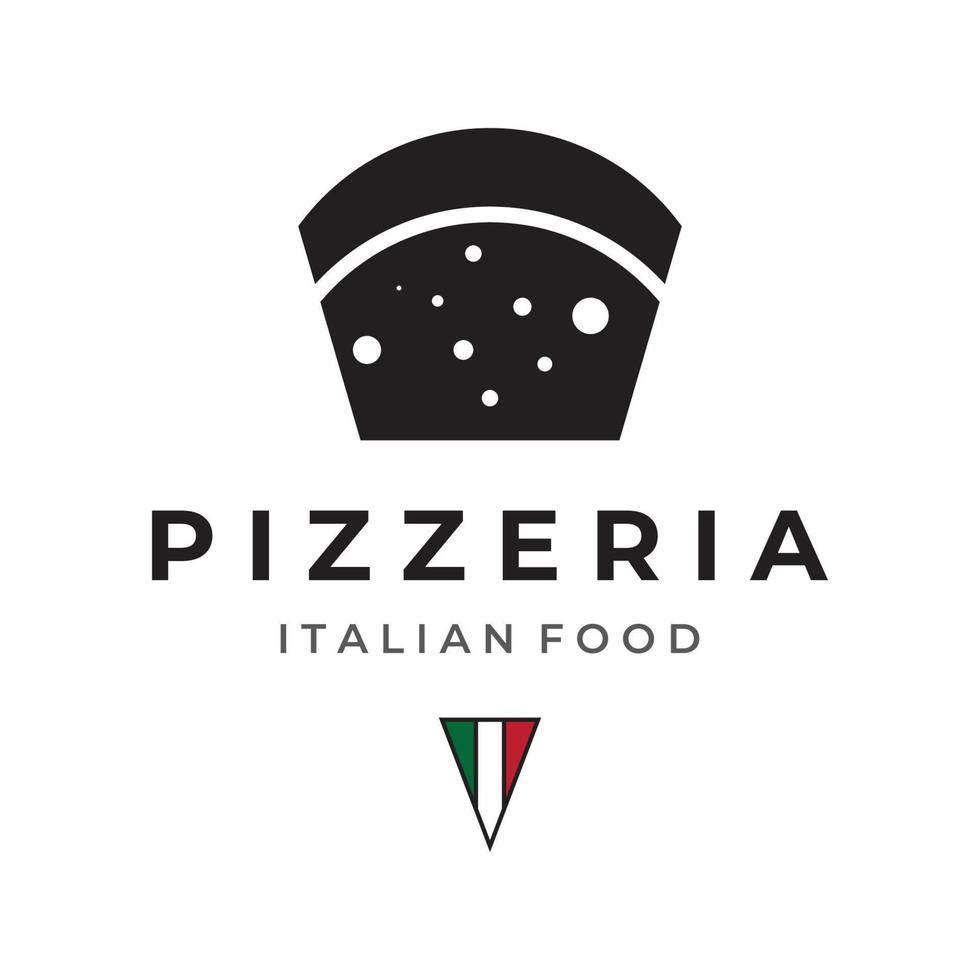The image features a stark white background and prominently displays a stylized, partial slice of pizza rendered in black. The pizza slice exhibits a unique design: its crust is solid black with a thin white line separating it from the body of the pizza. The body itself is adorned with variously-sized white circles, suggestive of pepperoni and cheese toppings. Below this artistic depiction, the word "Pizzeria" is prominently inscribed in bold black letters, accompanied by the phrase "Italian Food" in a slightly smaller black font. Adjacent to the text, a small triangular icon showcases the vibrant colors of the Italian flag—green, white, and red—adding an authentic touch to the overall theme.